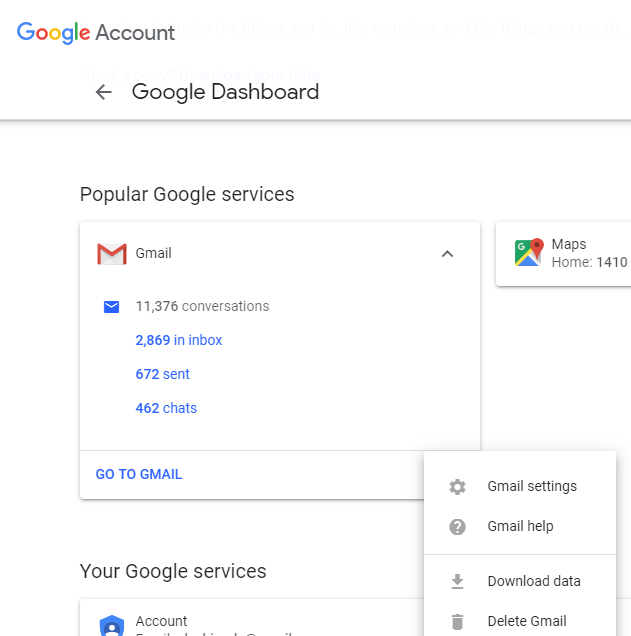The image depicts a Google Account Dashboard page. The top left corner prominently displays "Google Account" with "Google" rendered in blue, red, yellow, and green, and "Account" in gray. Directly below, a navigation indicator features a left arrow icon followed by "Google Dashboard." A horizontal line separates this header from the main content.

Under the section titled "Popular Google Services," the first item listed is "Google Mail," accompanied by an envelope icon. To the right is an upward caret, indicating a dropdown has been expanded. This reveals detailed statistics: "11,376 conversations," "2,869 inbox," "672 sent," and "462 chats." Below these statistics, a blue link reads "Go to Gmail."

Further down, there is a section labeled "Your Google Services." The visible portion shows "Account" at the top, but the rest is cut off. On the right side of the page, partially visible text shows "Maps Home" with a number, "1410," but it is also cut off. Additionally, a pop-up window lists various options related to Gmail, including "Gmail settings," "Gmail Help," "Download data," and "Delete Gmail." This text is gray, set against a white background consistent with the rest of the page.